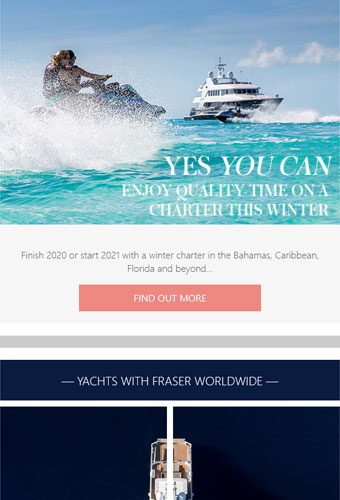The image appears to be an advertisement. At the top, there is a vibrant picture of people riding a jet ski with a boat visible in the background, evoking a sense of adventure and leisure. Overlaid on the image is the text: "Yes, you can enjoy quality time on a charter this winter."

Below the main image, there is a gray rectangle containing promotional text that reads: "Finish 2020 or start 2021 with a winter charter in the Bahamas, Caribbean, Florida, and beyond."

Adjacent to this, there is a salmon-colored rectangle with the call-to-action text: "Find out more."

The sections are separated by a thin white line, followed by a darker gray line and another thin white line beneath it. Further down, a dark blue rectangle with the text "Yachts with Fraser worldwide" in white lettering is prominently displayed.

Towards the bottom of the image, although it is partially cropped, there is an aerial photo showing the top view of a yacht, providing a glimpse of the luxurious experience being advertised.